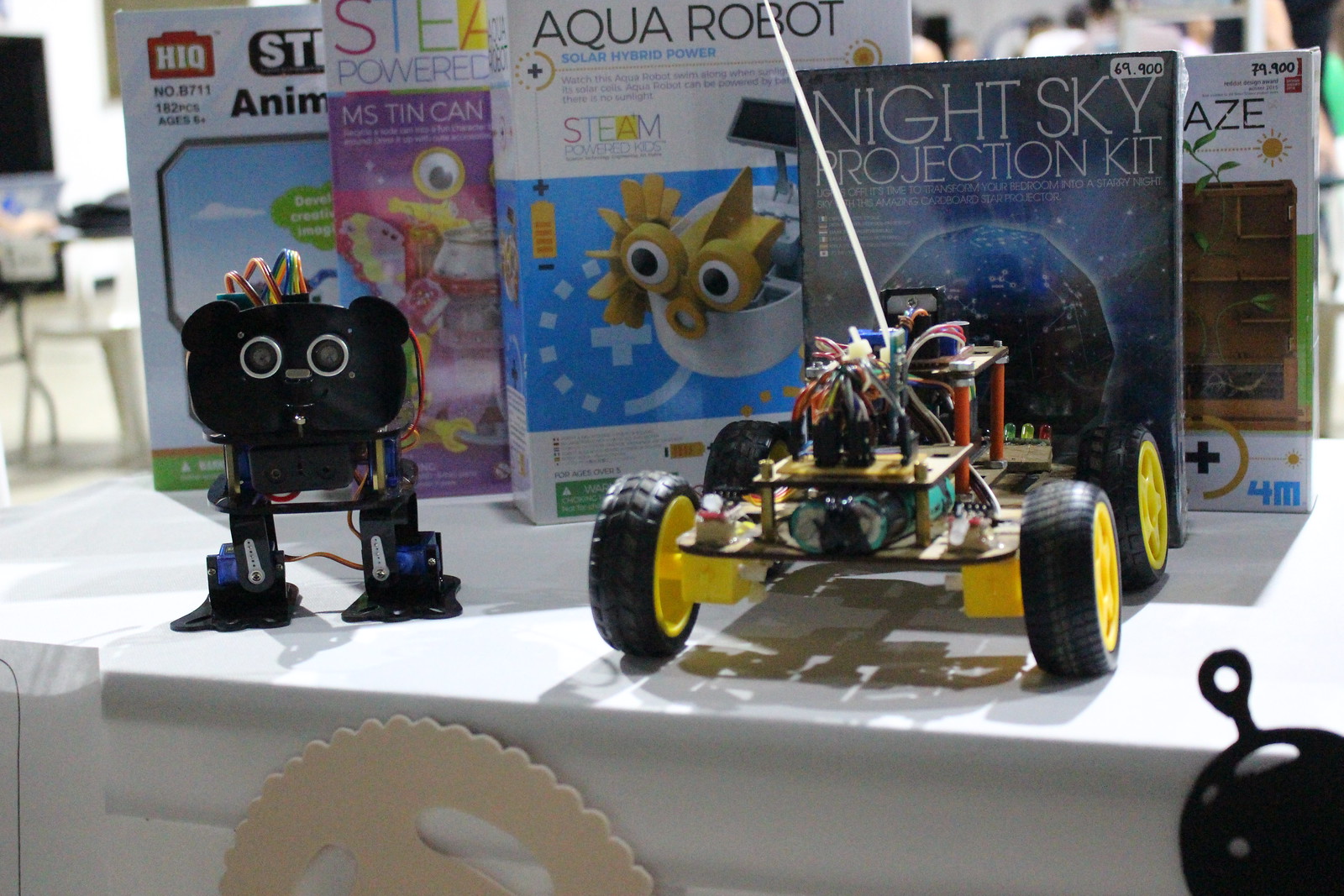The photograph captures a table adorned with a white tablecloth, showcasing an array of toys prominently displayed in an indoor setting. On the table sits a bipedal black robot, characterized by wires protruding from its head, two small circular eyes, and various exposed mechanical components. To its right is a four-wheeled RC car, notable for its antenna and visible internal circuitry including wires and battery components. 

In the background, a collection of boxes, primarily featuring construction toys and science kits aimed at children, is partially visible. Among these, the most prominent are the "Night Sky Projection Kit," displaying a globe surrounded by stars and priced at $9, and the "Aquarobot Solar Hybrid Power" kit, depicted on a white box with an image of a robot fish. Some of the other boxes are obscured, but hints of additional scientific project kits are evident, with another package featuring the letters "A-Z-E" and a price of $79 visible.

Near the edge of the table, there is a cut-out resembling a gear and a piece of paper to its left, adding a further touch of scientific exploration and DIY project ambiance to the scene.